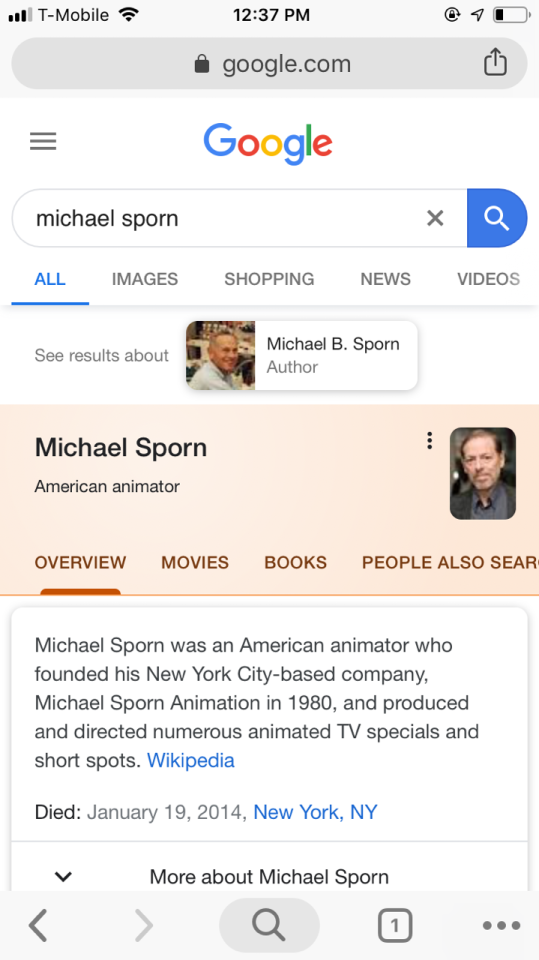A digital screenshot captures search results for "Michael Sporn" on Google. The interface shows three out of four full bars for T-Mobile signal strength, Wi-Fi connected, the time at 12:37 PM, and a low battery icon. At the top, the Google logo and search bar display the query "Michael Sporn." Navigation tabs for "All," "Images," "Shopping," "News," and "Videos" are visible, with "All" being currently selected. Below, a beige header labeled "Overview" presents various result categories including "Movies," "Books," and "People also search."

The primary result details Michael Sporn as an American animator with an adjacent photograph. The text notes that Sporn founded the New York City-based Michael Sporn Animation in 1980 and was known for creating numerous animated TV specials and short films. The Wikipedia link provides additional information. Key biographical details include his date of death, January 19, 2014, in New York, NY, both hyperlinked for more details. A dropdown at the bottom suggests "More about Michael Sporn."

Additionally, the bottom menu contains navigation buttons - a clickable back arrow, a grayed-out forward arrow, a search button, a home icon within a square, and a three-dot menu on the right.